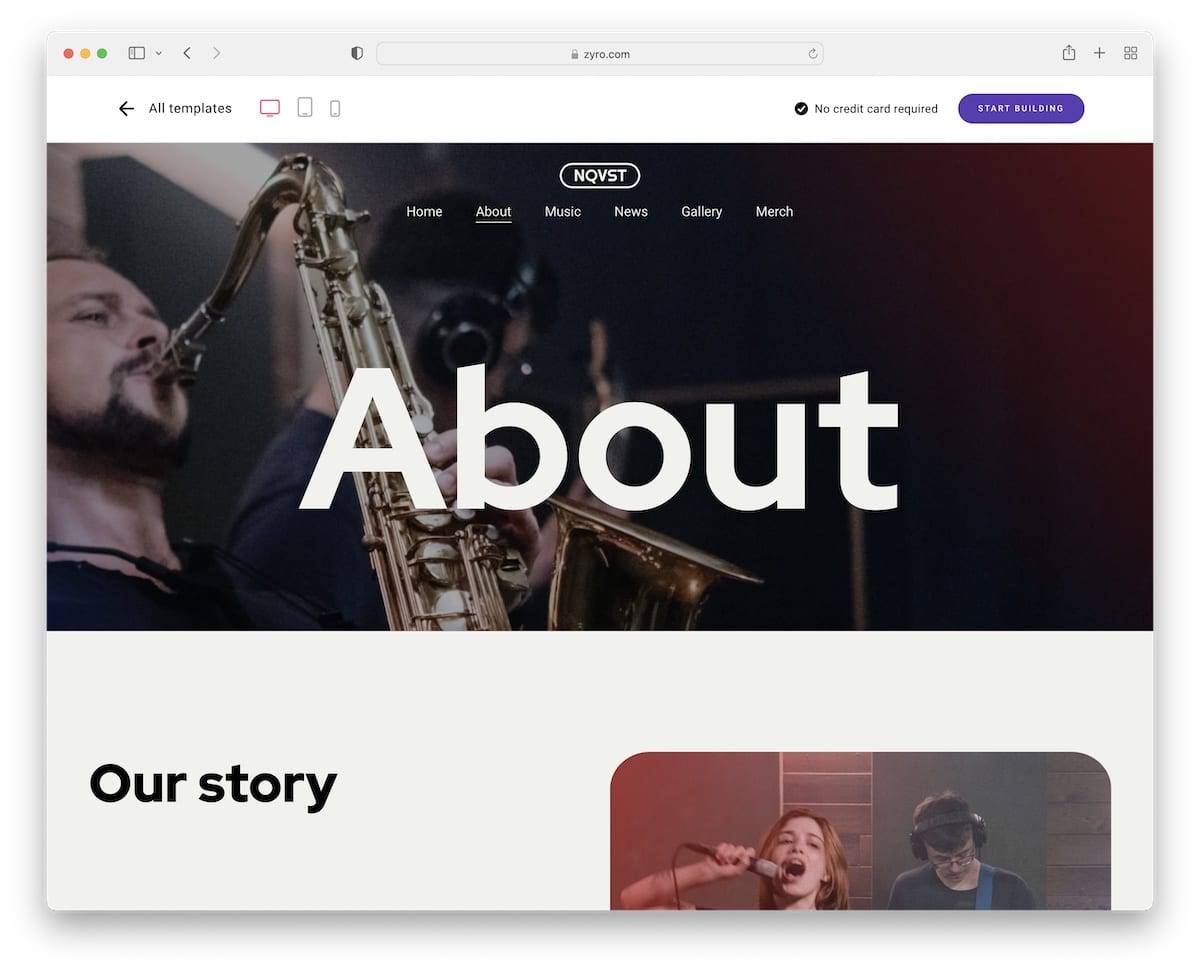The image displays a screenshot of someone viewing a website on a macOS browser, identifiable by the red, yellow, and green close buttons in the upper left-hand corner. The website URL reads "zyro.com," featuring various webpage elements. 

At the top, there is a selection of buttons within the browser's chrome, including navigation options and tools. Below, the page title "All Templates for Website" is present, with options to view templates tailored for desktop screens, tablets, and phones. There is a prominent purple button labeled "Start Building" and a note indicating "No Credit Card Required."

Further down, the website menu appears in a capsule shape, with options labeled "Home," "About," "Music," "News," "Gallery," and "Merch." The "About" section is underlined, indicating it is currently selected. This area features a large, bold white title that reads "ABOUT," overlaid on a background showing a man playing a saxophone and another person, possibly playing a guitar, wearing a headset. This image has a dynamic red light leak effect on the right side, blending into the background.

Accompanying the section title "OUR STORY," there is a large photograph on the right side showing a woman singing into a microphone. Next to her is a man—likely the same person from the previous image—wearing glasses and a headset. Both photos have distinct visual elements: the first image is slightly obscured from a side angle, while the second is a clear, front-facing shot. The man in both images wears similar-colored t-shirts, adding visual continuity.

The screenshot is framed with a heavy drop shadow, isolating the browser window against a plain white background. This reinforces the focus on the website content, emphasizing its interface and design elements.